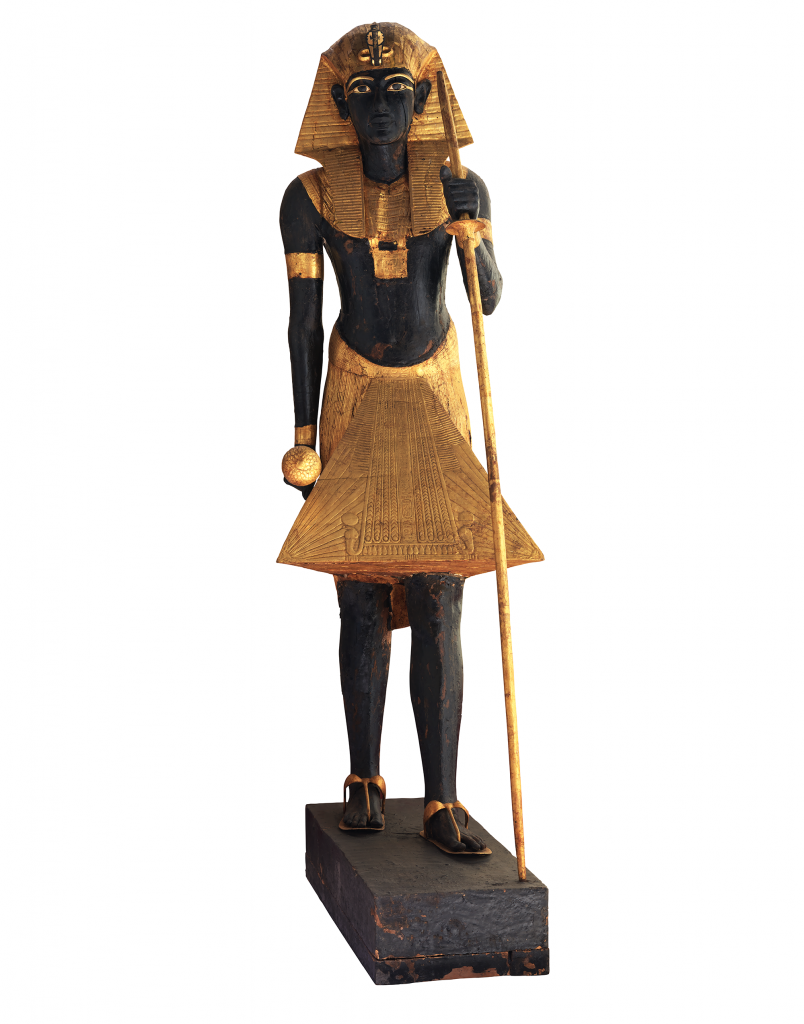The image features a detailed miniature sculpture of an Egyptian leader, standing on what appears to be a silver or granite block. The figure is predominantly black in color and exudes an aura of ancient Egyptian royalty. The leader is depicted holding a long, thin staff in their left hand, which extends vertically to the ground, with the elbow bent at an angle slightly greater than 90 degrees. In the right hand, positioned at their side, the figure holds a round object. 

The sculpture showcases traditional Egyptian attire, including a golden head covering that drapes along the shoulders, reminiscent of the times of mummies. The leader sports a golden band around the left shoulder and matching gold wristbands. Though the upper torso appears bare, the attire includes a distinctive skirt that flares outward in a three-dimensional, triangular shape. The figure wears thin golden sandals, adding to the regal appearance.

Additional golden details accentuate the sculpture, with golden eyebrows and highlights around the eyes, bringing a striking contrast to the otherwise black features of the statue.